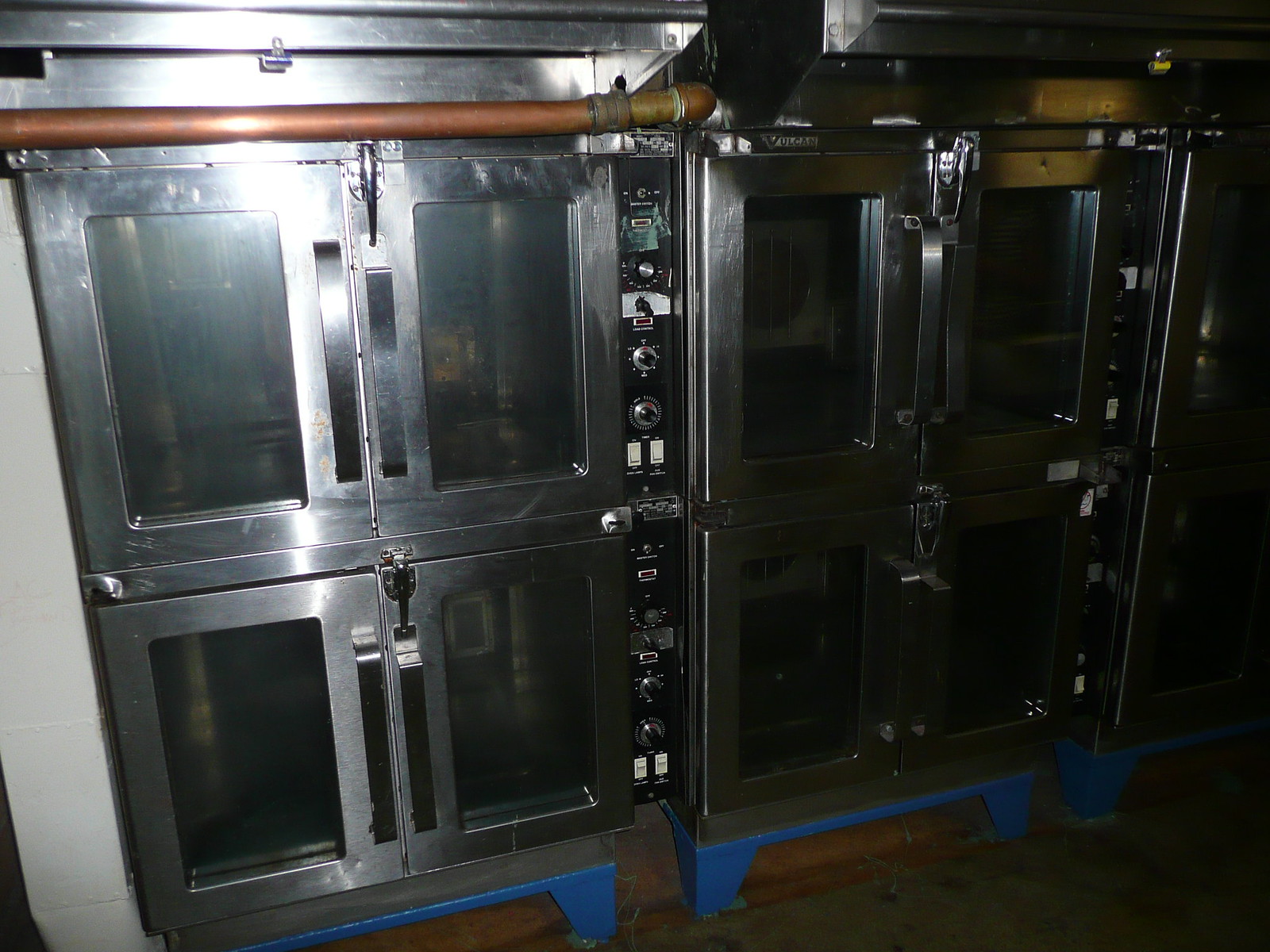This photograph showcases a series of industrial ovens, each with a sleek silver tone finish. The units are arranged in stacks of two, and the image captures at least four complete ovens along with parts of additional ones. A distinctive copper pipe runs horizontally across the very top of the leftmost oven. Each oven features double-doored fronts with clear tempered glass windows for visibility. The doors, fitted with central silver handles, open outward from the middle. On the right side of each unit, there is a black control panel adorned with numerous dials and knobs arranged vertically. Below the ovens, sturdy blue metal legs support the weight of the units, further reinforced by a black base that connects to the legs. The clean, industrial design suggests the ovens are likely used for specialized commercial or industrial baking processes.